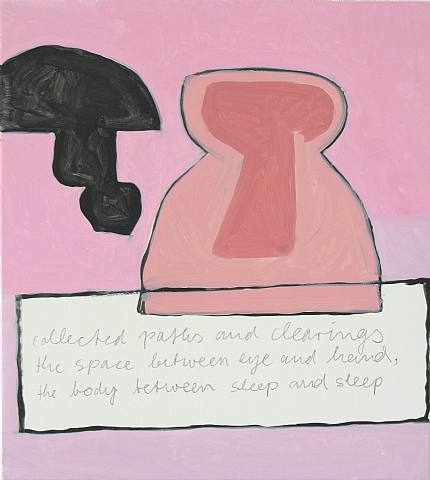This image appears to be an abstract painting with a background in a light to medium shade of pink. On the left side near the top, there is a black abstract figure resembling a mushroom, with a rounded top and a trailing bottom that extends to the right. To the right of this, there is a light pink shape, outlined in black with a darker pink center, which some suggest resembles either a bag of money or the lower body of a woman starting from the breast area to the thighs. At the bottom of the image, there's a white rectangle with cursive text. The text appears to read: "collected parts and clearings, the space between eye and hand, the body between sleep and sleep." This descriptive and somewhat poetic caption offers insight into the abstract nature of the artwork.